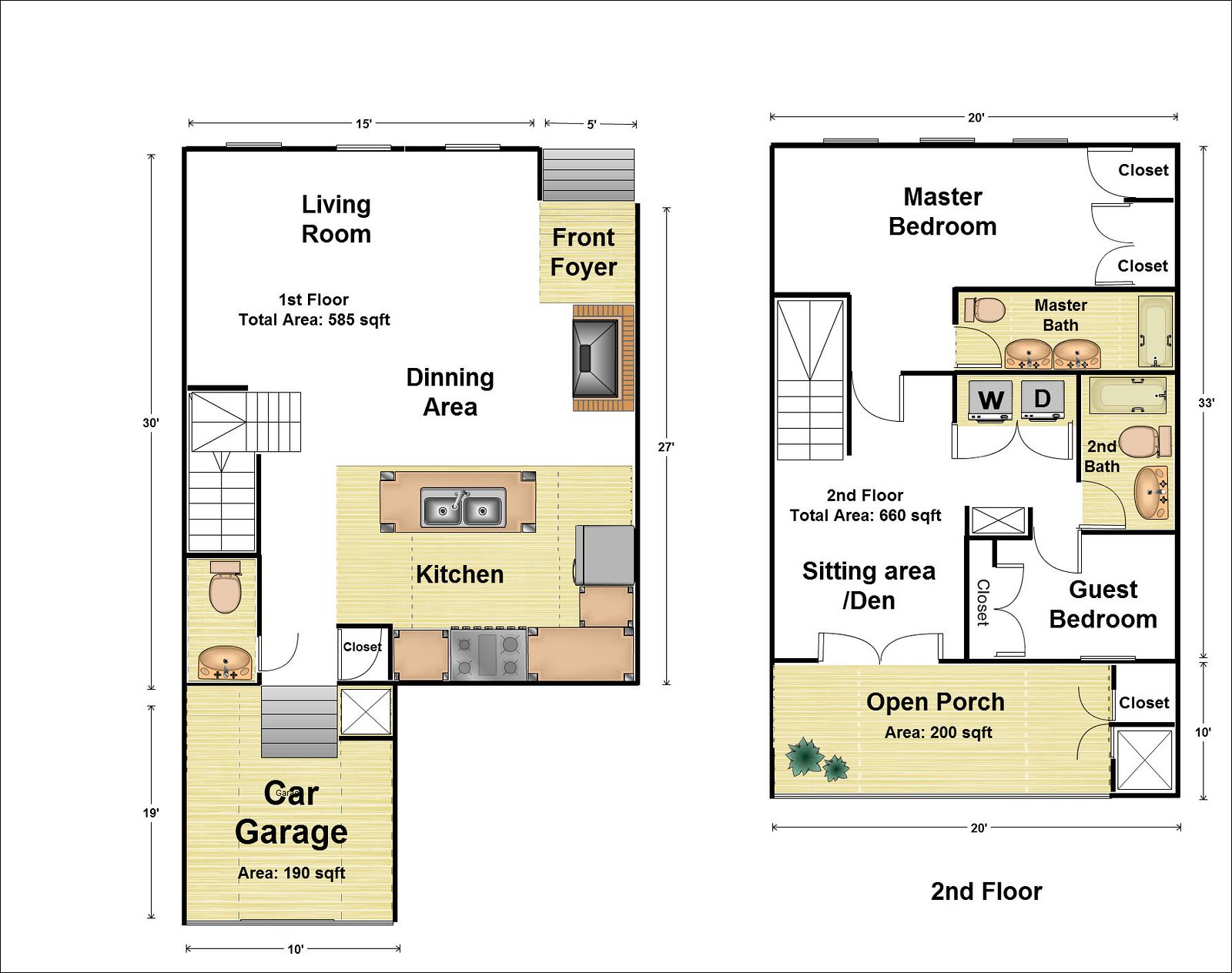This detailed architectural layout presents the floor plans for a two-story house, complete with precise measurements and room specifications. 

**First Floor:**
Upon entering from the 190-square-foot garage positioned at the bottom center of the floor plan, one encounters a well-organized layout. Directly to the left is a half bathroom, and immediately to the right is a closet for storage. Moving further upward on the plan, the right side reveals a fully equipped kitchen, featuring essential appliances such as a stove, sink, refrigerator, and ample cabinet space for storage. Adjacent to the kitchen is a dining area, seamlessly leading into the spacious living room, which extends into the front foyer, welcoming guests.

**Second Floor:**
Ascending to the second floor, one will find an open porch that provides an inviting outdoor area. Inside, a cozy sitting area or den serves as a versatile space for relaxation or work. The second floor also includes a guest bedroom and a laundry room equipped with a washer and dryer, ensuring convenience. A full bathroom services this floor, offering comprehensive amenities compared to the half bath downstairs. The master bedroom is the highlight, boasting two separate closets for ample storage and a private master bath for added luxury.

In summary, this house features two bedrooms, two and a half bathrooms, a fully equipped kitchen, a living room, a dining area, a garage, and an open porch, all thoughtfully designed to combine function and comfort.